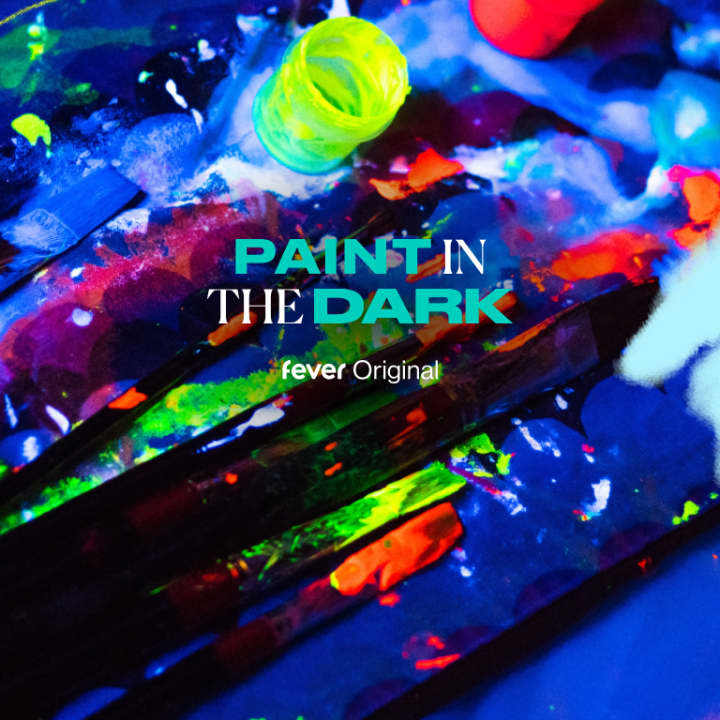The image appears to be a vibrant and artistic cover, potentially for an album, a book, or an advertisement for an activity. It features a visually striking blend of neon, gold, and dark colors, including blues, oranges, fluorescent greens, pinks, purples, and reds, all splattered and smeared in an abstract, backlit design that creates a glowing effect. The composition is a square canvas with no distinctive border, showcasing a lively mix of textured colors. Centrally located text reads "PAINT IN THE DARK" with "paint" in lighter blue and "in the" in white, while "dark" is in green. Beneath this, in smaller white lettering, is the phrase "FEVER ORIGINAL." Additionally, the image includes elements like paintbrushes with neon orange paint and a paint palette, enhancing the dynamic and colorful appeal.